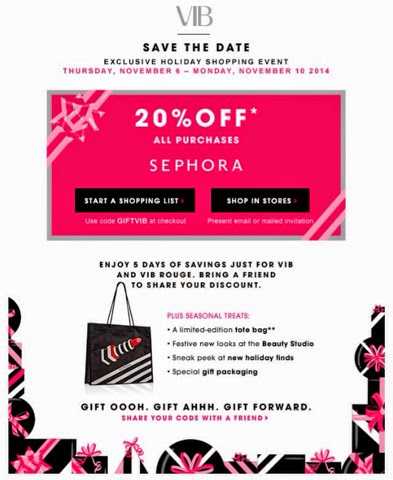The poster advertises an exclusive holiday shopping event hosted by Sephora for VIB (Very Important Beauty Insider) members. The event is scheduled from Thursday, November 6th, to Monday, November 10th, 2014. Prominently displayed on the poster is an eye-catching offer: "Save the Date - 20% off all purchases at Sephora." Two interactive black buttons prompt viewers to start a shopping list or shop in stores.

Scrolling down, the poster highlights the benefits of this five-day shopping extravaganza, emphasizing savings exclusively for VIB and VIB Rouge members. It encourages members to bring a friend to share the discount and enjoy seasonal treats. An image of a limited edition tote bag with stylish black and white stripes and a clever lipstick design is showcased, indicating the special item members can receive. Additional perks include festive new looks at the beauty studio, a sneak peek at new holiday products, and special gift packaging. This comprehensive invitation is designed to enhance the holiday shopping experience for Sephora's loyal customers.